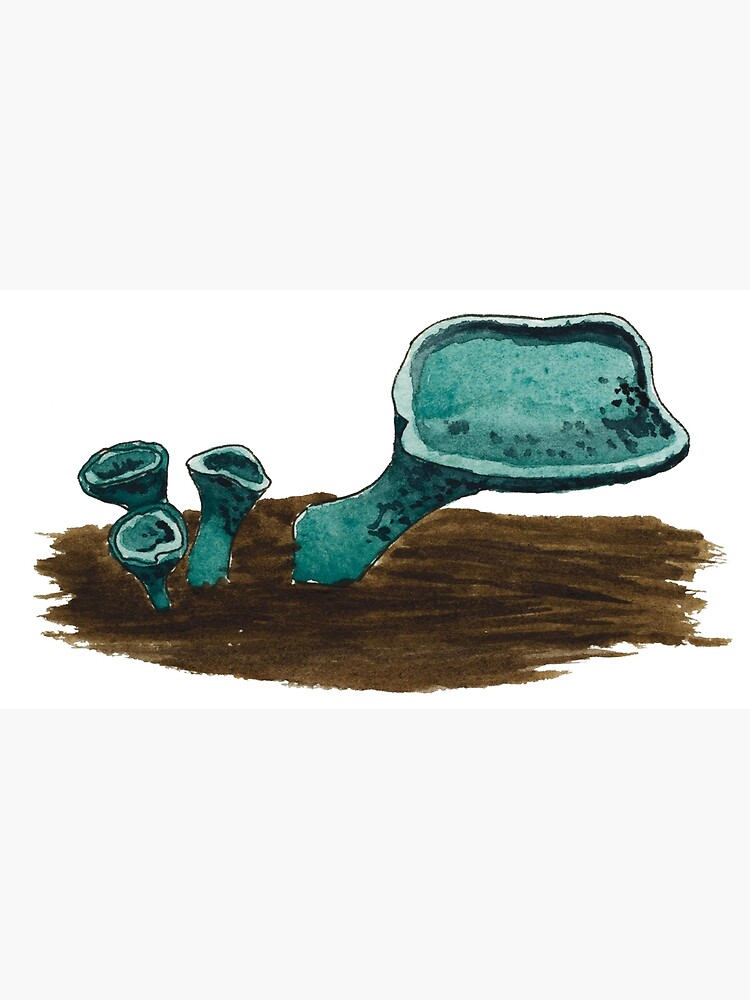This detailed illustration depicts an imaginative scene featuring four bluish-teal mushrooms emerging from a flat patch of dark brown soil. The background is stark white, emphasizing the contrast between the earthy tones and the surreal colors of the fungi. The most prominent mushroom, positioned slightly towards the right side of the patch, boasts an oblong head with a deep indentation and a long, sturdy stalk. It's notably larger than its companions and leans slightly to the right. 

On the left side of the dirt patch, three smaller mushrooms cluster together, their shapes suggesting they might grow to resemble the larger one. These mushrooms also have oblong, indented heads and long stalks, with the smallest mushroom facing forward while the other two reach upward as if striving toward sunlight. The teal-blue hue with subtle speckles adds an otherworldly quality, reminiscent of sea anemones, suggesting these might be mushrooms from an alien planet, as they certainly don't match any known earthbound fungi. The soil is uniformly colored with visible brush strokes, devoid of texture, which contrasts with the intricate detailing of the mushrooms. This distinct, almost oceanic portrayal gives the artwork a captivating, alien aesthetic.